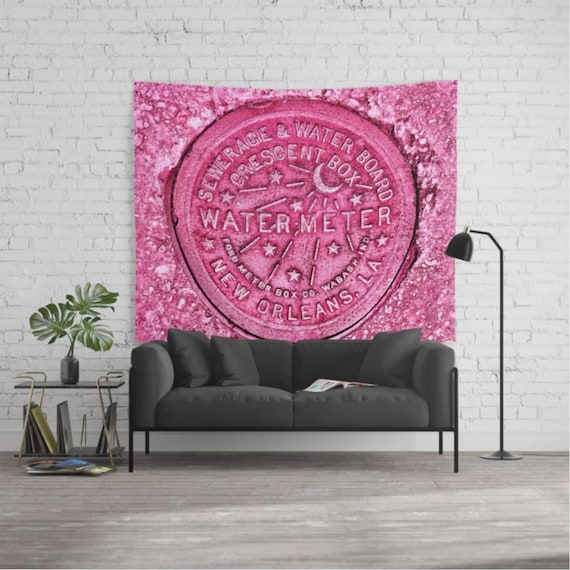The photograph captures an indoor setting, likely in a warehouse-styled New York apartment, featuring a gray two-seater couch with a black metal frame on a gray wooden floor. The backdrop is a white-painted brick wall adorned with a large pink tapestry, which is a blown-up image of a water meter cover. The text on the tapestry reads "Sewage and Water Board, Crescent Box, Water Meter, New Orleans, Louisiana." To the left of the couch is a small metal side table with vinyl records or books on the bottom shelf and a black vase holding a Monstera plant with three leaves. On the right side of the couch, there's a black metal lamp. The overall color scheme is muted and industrial, with the pink tapestry providing the only vibrant splash of color in the room.